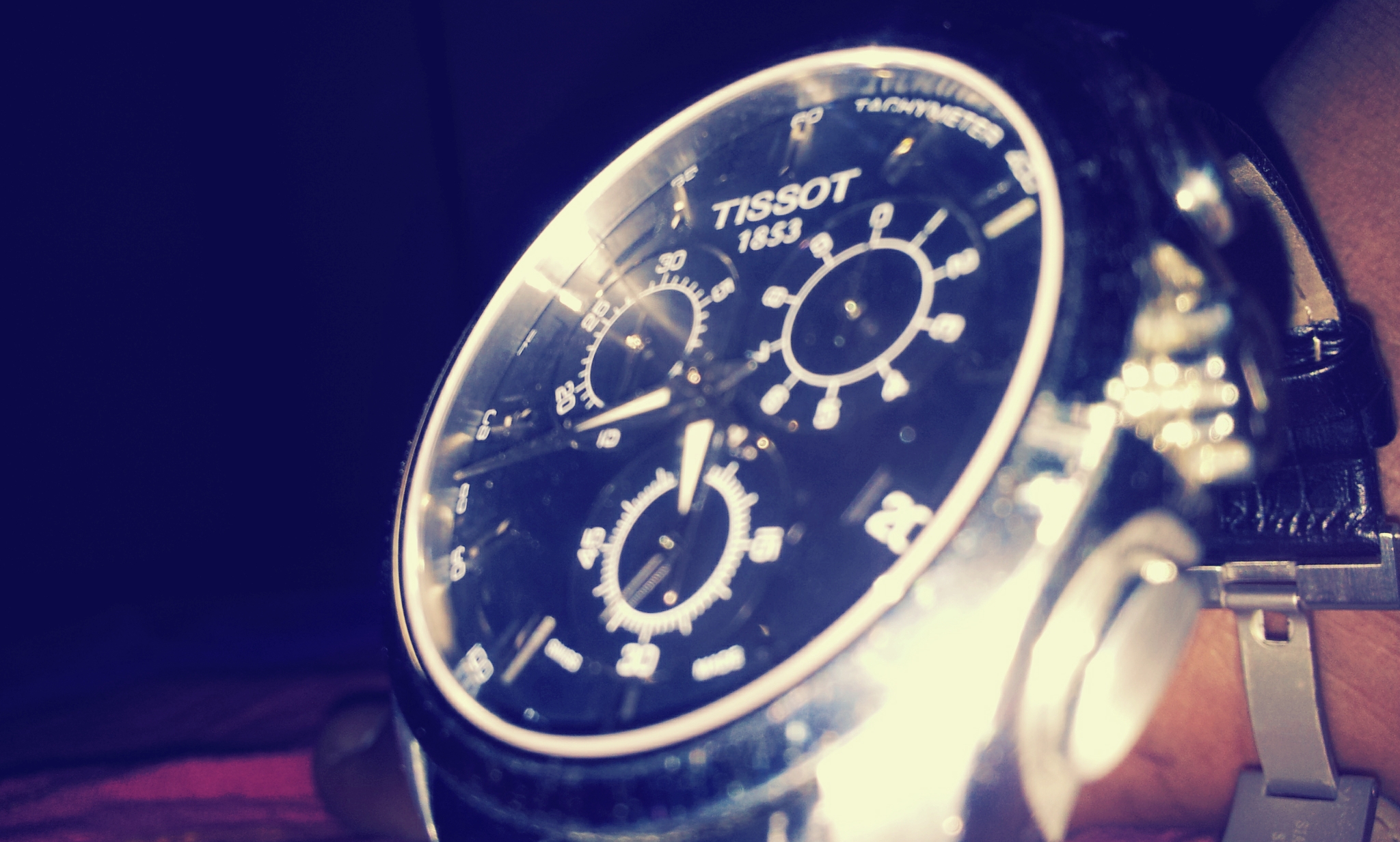This detailed and descriptive caption might suit your needs:

"The image showcases an elegant circular wristwatch with a pristine white outer casing. Prominently displayed at the top of the watch face, where the 12 o'clock position is typically found, is the brand name 'Tissot' followed by the year '1853.' The watch face is intricately designed, featuring several smaller sub-dials that function as odometers, marked with increments of 5, 10, 15, 20, 25, 30, and 45. Each sub-dial is equipped with its own set of hands for precise timekeeping. Underneath the watch, a glimpse of the wearer's skin is visible, along with a metallic buckle that secures the watch snugly around the wrist."